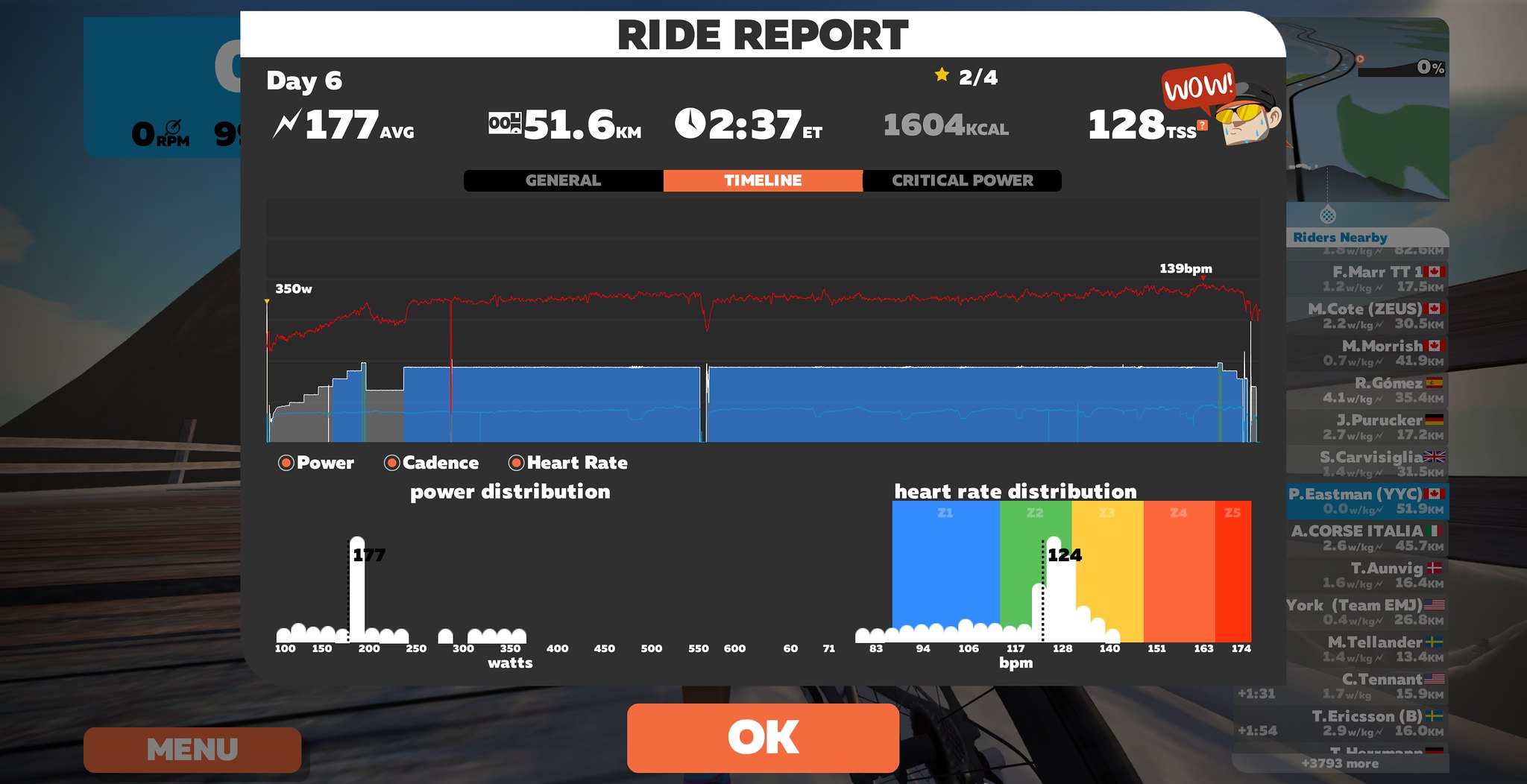The image is a screen grab from a computer showing a detailed bar chart of a health tracker, specifically from a bicycle ride. At the top, a white banner with black text reads "Ride Report." Below this banner, a series of metrics is displayed against a black background with white text. From left to right, the data includes "Day 6," indicating the continuation of a program, with an average value of "177," a distance covered of "51.6 KM," and an estimated time of "2:37" (likely 2 hours and 37 minutes). It also shows "1604 Kcal" burned and a Training Stress Score (TSS) of "128."

To the right of this data, there is a cartoonish image of a sweaty man wearing yellow glasses, accompanied by a red speech bubble saying "Wow!" in white font. The bottom part of the screen contains multiple colored charts and graphs. A red line traces over bar graphs representing different metrics such as power, cadence, and heart rate. Another section highlights "watts" with a scale ranging from 100 to 600. Adjacent to this, there's a heart rate distribution graph. Additional details include orange tabs labeled "OK" and "Menu," and a section labeled "Riders Nearby," suggesting an interactive element possibly linked to a virtual race or a Peloton-style course. A bicycle tire at the bottom of the image further suggests this is a cycling-related health tracker.